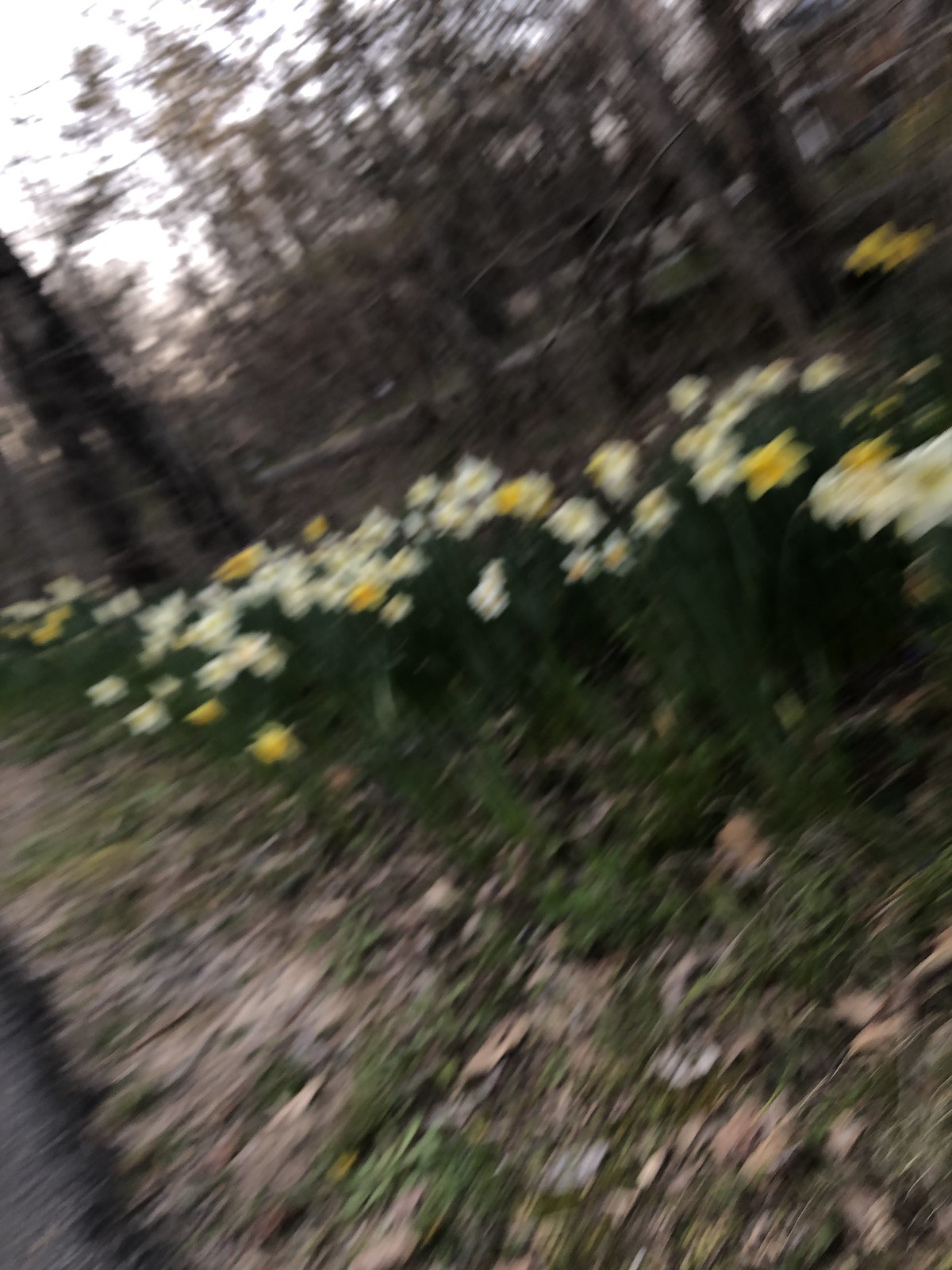In the photograph, a blurred outdoor scene captures an array of spring blossoms, likely narcissus or jonquils, predominantly in shades of yellow and pale yellow. These flowers stretch nearly horizontally across the image. In the foreground, the ground is strewn with dead leaves interspersed with patches of greenery. Midway through the scene, on the far right, a house can be faintly discerned. A backdrop of trees, some adorned with sparse foliage and others appearing rather bare, adds depth and texture to the composition. In the bottom left corner, a grayish strip suggests the presence of a road or pathway, adding a subtle contrast to the natural elements in the scene.